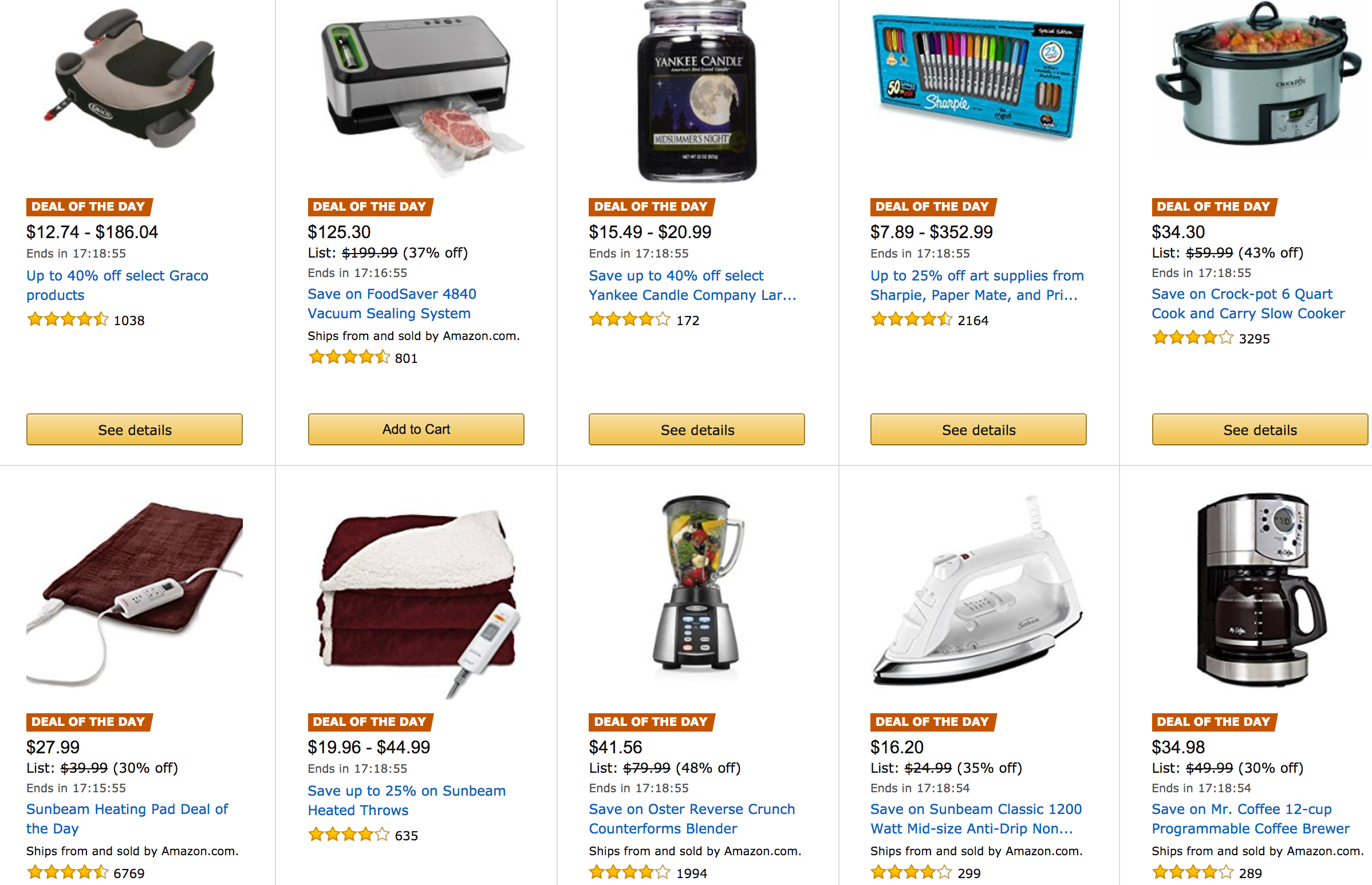This is a detailed screenshot of the Amazon website, characterized by its signature yellow, orange, and white color scheme. The page showcases various "Deal of the Day" products, each marked with an orange banner indicating the promotion.

### Top Row:
1. **Car Seat and Baby Seat**: Positioned on the far left, this product is a car seat intended for infants or young children, to be installed in the back seat of a vehicle. The price range is listed as $127.4 to $186.04.
2. **Oven or Food Dehydrator**: Next to the car seat, this item appears to be an oven or a similar kitchen appliance. The image shows a piece of raw meat, hinting at its culinary purpose, with a price of $125.
3. **Black Bottle**: This product is a black-colored bottle of unknown contents, placed in the center of the top row.
4. **Marker Set**: To the right of the bottle, there’s a colorful set of markers, designed for drawing or coloring.
5. **Rice Cooker or Slow Cooker**: On the far right of the top row, this appliance appears to be a rice cooker or slow cooker, used for preparing meals with convenience.

### Bottom Row:
1. **Digital Board with a Meter**: Starting from the left, this item is an electronic board equipped with a meter, possibly for technical or engineering use.
2. **Bag**: Next to the digital board, there is a bag, the specific type or purpose of which is not clear from the image.
3. **Thermometer-like Device**: To the right of the bag, there is an instrument resembling a thermometer, likely used for temperature measurements.
4. **Blender**: Positioned fourth from the left, this appliance is recognizable as a blender, ideal for making smoothies or puréeing ingredients.
5. **Steam Iron**: On the far right, there is an iron, presumably for clothing, to remove wrinkles and creases.
6. **Coffee Maker**: At the very end of the bottom row, there is a coffee maker, perfect for brewing fresh coffee at home or in an office.

Overall, the screenshot displays a variety of products ranging from household appliances to personal care items available at discounted prices on Amazon.